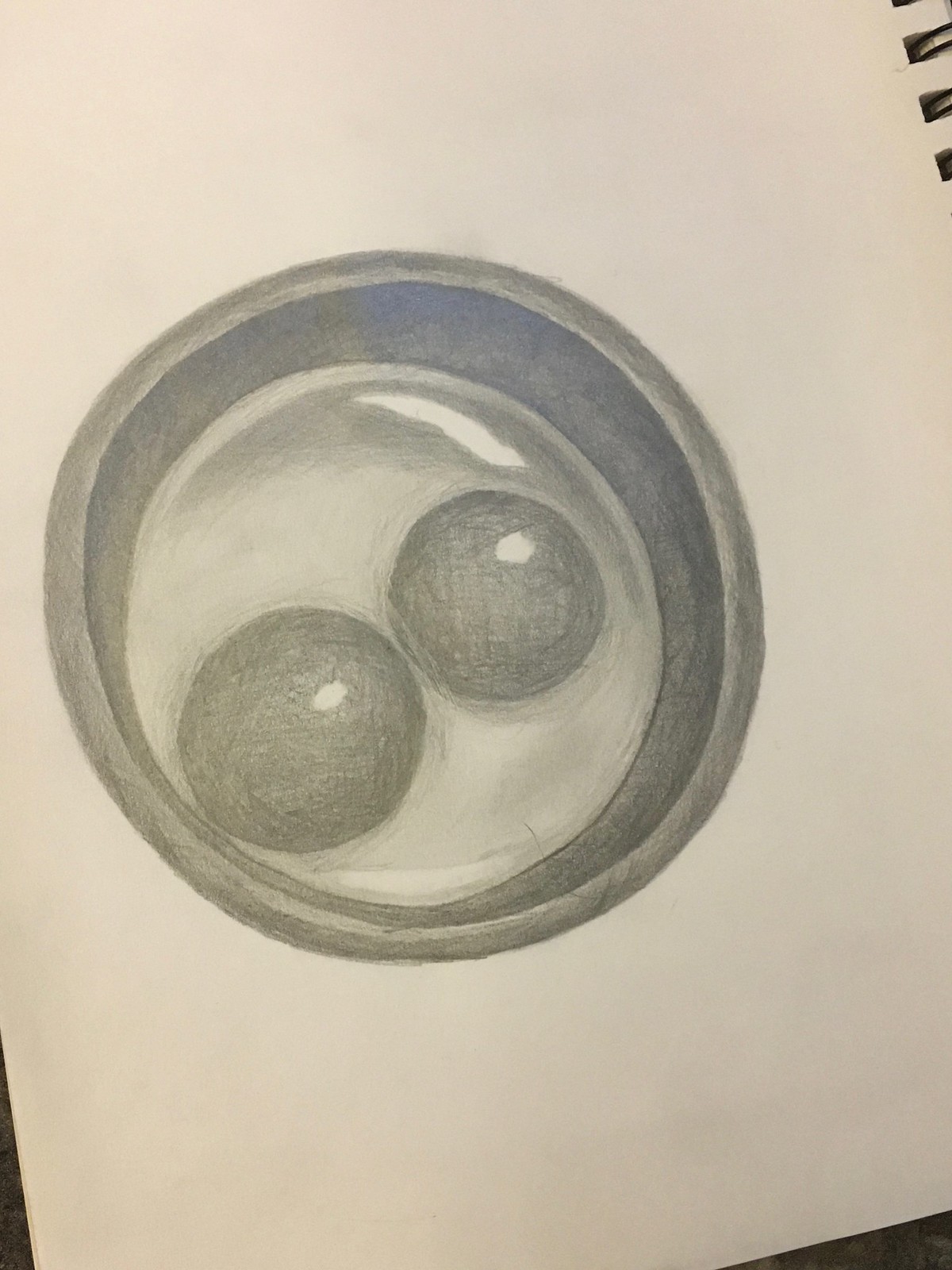The image features a detailed drawing centered on a rectangular piece of white paper. The paper is part of a spiral-bound notebook, with the silver-colored spiral visible in the top right corner, showing four holes. The drawing itself is circular and rendered entirely in black ink, maintaining a monochromatic black-and-white contrast. Within the circular drawing, two prominent round black circles are situated in the middle, adding to the intricate design. There are no other elements or distractions in the image, making the drawing the sole focus.